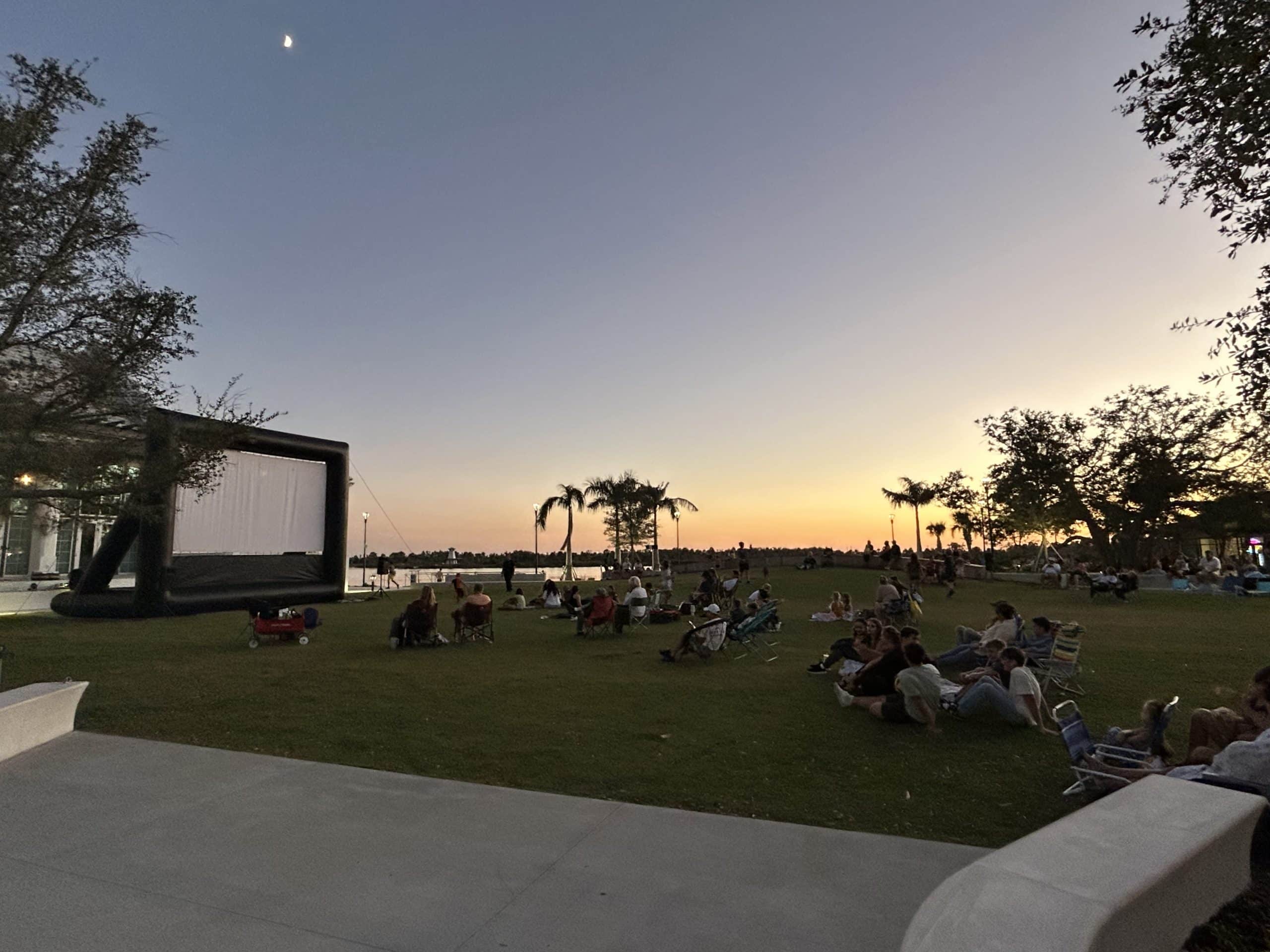The image captures a tranquil, tropical evening in a small city park featuring a large, manicured field, reminiscent of a southern Florida setting. The scene is set just past sunset, with the sky transitioning from deep blue to hues of yellow and orange, and a sliver of the moon visible in the upper left corner. In the foreground, attendees are gathered facing a large, inflatable projector screen bordered in black, indicating an outdoor movie or video presentation is about to start. The crowd is diverse, consisting of people sitting on blankets, lawn chairs, and in little red wagons. Children play nearby, contributing to the relaxed, communal atmosphere. Palm trees and leafy trees frame the scene, with a bit of a lake and possibly an ocean cove visible in the background, enhancing the peaceful, tropical ambiance as dusk settles in.